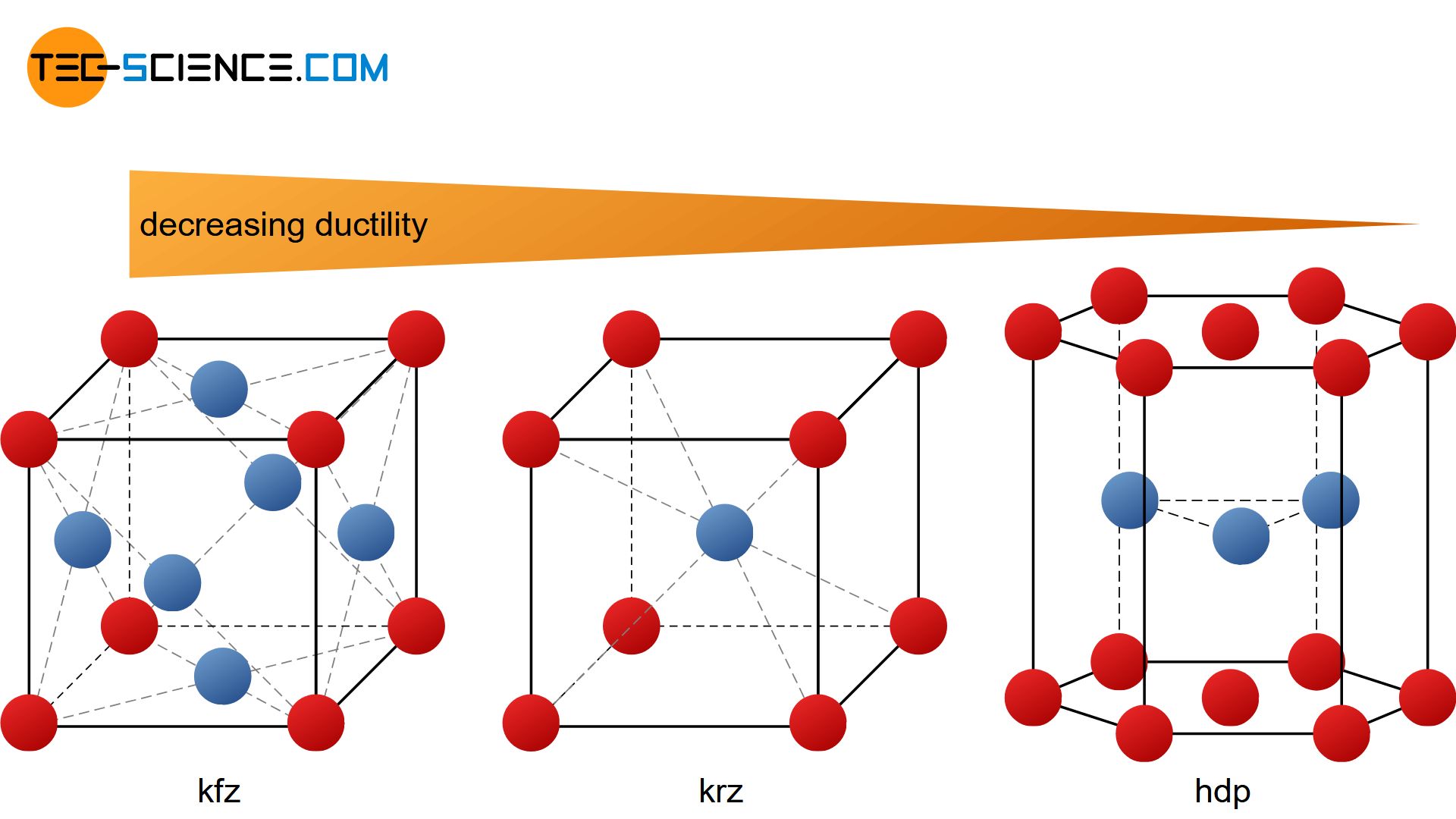The image is a rectangular chart with a white background. The top and bottom sides are twice as long as the left and right sides. In the top left corner, there's an orange circle with black text that reads "tech." Outside the circle, there is a dash followed by "science.com," where the 'S' in "science" and "com" are in blue.

Below that, there is an orange triangle that spans the entire width of the image, tapering to a point as it moves from left to right. Inside the triangle, in black lowercase letters, is the text "decreasing ductility."

The bottom of the image features three molecular-like diagrams arranged horizontally. The first diagram on the left is labeled "KFZ" and is square-shaped with red circles at each corner. Inside, it contains six blue circles and additional red circles connected by dotted gray lines. The middle diagram, labeled "KRZ," also has red circles at the corners and includes one blue circle and one red circle within, also connected by dotted gray lines. The rightmost hexagonal diagram, labeled "HDP," features red circles on its vertices and a blue circle with a triangular arrangement inside. These shapes depict decreasing ductility and the interconnected nature of different elements, with blue and red circles representing various atomic components.